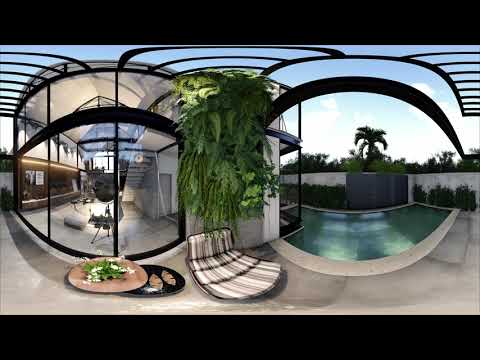In this detailed panoramic fisheye image, we observe a sophisticated outdoor and indoor setting of a house. To the right, a large swimming pool curves gracefully like a rainbow, bordered by lush greenery and hedges. Beyond the hedges, there is a stone wall with a palm tree and other verdant foliage visible in the background. 

Moving left from the pool, you reach the beginning of the house where a modern metal frame structure stands in front. Within this structure, a white floor is prominent, and a black-and-white striped seating area (possibly a bed-like sofa) occupies the center. Above this seating area, an abundant, bushy green plant dangles down, adding a touch of nature to the sleek design.

There's a curved and arched motif in the black, bold, and thick lines that run across the image, creating horizontal stripes and vertical lines that enhance the modern aesthetic. These lines frame the glass-enclosed room on the left side, through which we can see the white flooring, a staircase, and an interior lit from the top. In front of this glass room, a dining area is visible with a round beige dining table and a nearby small dining table with a plant placed on it.

Upon closer inspection, various objects are scattered around: a black and beige object on the ground, and plates with food (a brown plate with salad and a black plate with meat cutlets) suggesting a cozy, lived-in atmosphere. On the far left, stairs ascend, leading towards more unseen parts of the house, capturing the essence of modern, spacious, and intertwined indoor-outdoor living.